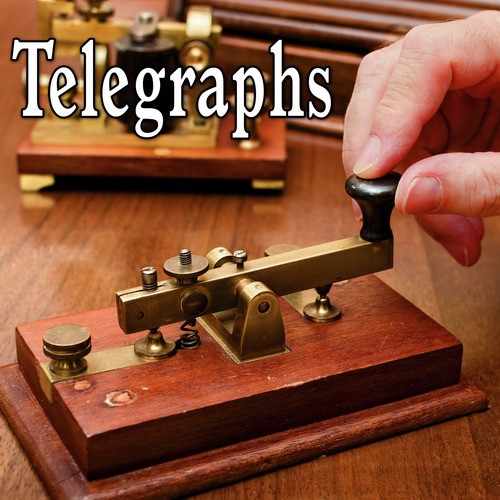The image depicts an antique telegraph device prominently labeled "TELEGRAPHS" in bold, white letters outlined in black at the top left. The telegraph sits atop a polished wooden table or desk. Central to the image is a hand partially visible on the right side, with its thumb, index, and middle finger gripping a small black knob attached to the device. This telegraph features a gold mechanism in the middle, likely made of brass, and is mounted on a dark brown rectangular base. In the background, another similar but larger telegraph device can be seen, also adorned with gold and black components. To the right of this background device, there's a brown object that appears to be a case or cover. The image captures the intricate details and craftsmanship of the telegraph components and their historical significance.